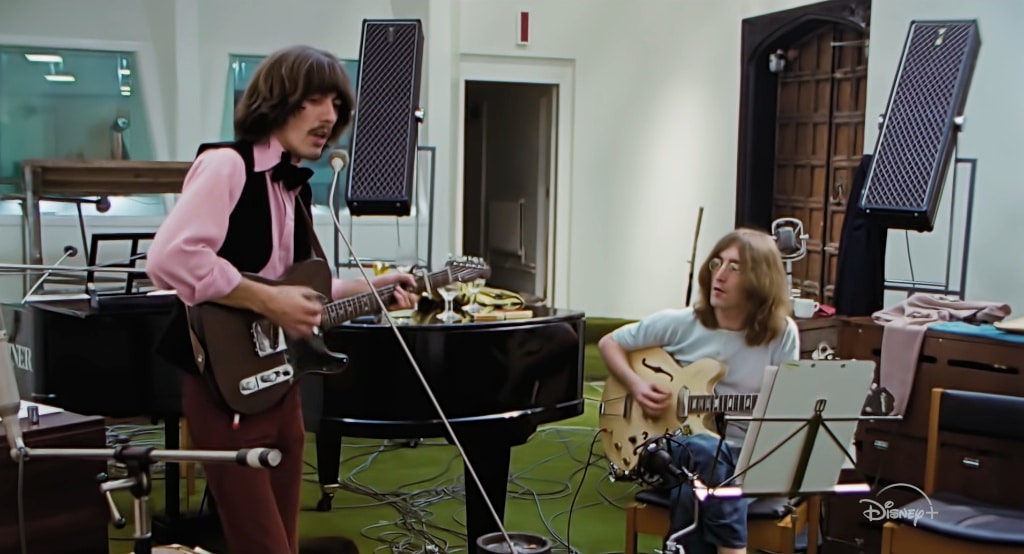This detailed photograph, likely from a home movie or documentary, features two young members of The Beatles, George Harrison and John Lennon, in a music studio. On the left side of the image, George Harrison stands holding a dark brown guitar. He is dressed in a pink long-sleeve shirt, black vest, and red velvet pants, with shaggy brown hair. John Lennon sits on the right side, cradling a larger, light cream electric guitar. He sports blue jeans, a white short-sleeve shirt with glasses, and longer blonde hair. The studio has a green floor and white walls, adorned with various microphones, a black baby grand piano with clear champagne glasses on top, and a music stand in front of John. The space's left side features glass windows, likely for musical engineers, and in the background middle, a door with a recording light. On the right edge of the image stands a pair of tall, double-wide wooden doors, emphasizing the studio's spaciousness.